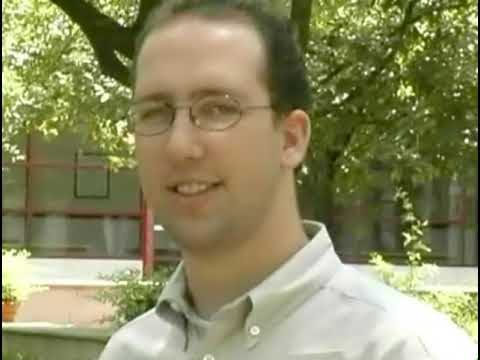This square photograph captures a smiling man outdoors in what appears to be an academic setting, perhaps a college or school. The man's face and shoulders are visible, and he is clean-shaven with a partially bald head, featuring short brown hair mostly at the back and sides. He wears oval glasses and a collared, button-down shirt that appears to be tan or gray. His smile reveals his top teeth, giving him a friendly expression.

In the background, there is lush greenery with trees, numerous branches, and green leaves. Some portions of a tan building with red railings are also visible, lending to the academic atmosphere. There is a potted plant with white flowers on a short stone wall in the lower left corner, adding more detail to the scene. The photograph, though somewhat blurry, captures the man centrally amidst this verdant outdoor setting, framed by a mix of natural and architectural elements.